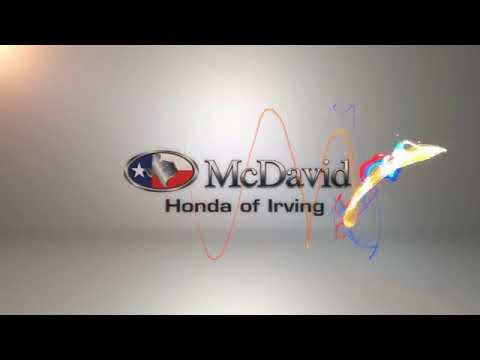The promo splash screen for McDavid Honda of Irving features a sophisticated silver and white gradient background, providing a sleek, modern feel. Dominating the left side, an oval emblem prominently displays the vibrant Texas flag, intricately bordered in silver, with a silver silhouette of the Texas state set within the flag. Positioned to the right of this emblem, the brand name "McDavid" is presented in a bold, silver and black font, with "Honda of Irving" aligned directly below in a smaller, black font. A dynamic visual element is introduced by an orange and yellow squiggle that traverses the center, creating arches over the McDavid Honda of Irving text, and culminates in a vibrant, mostly rainbow-colored splash. The upper left corner of the image subtly transitions into a lighter white shade, enhancing the overall gradient effect.